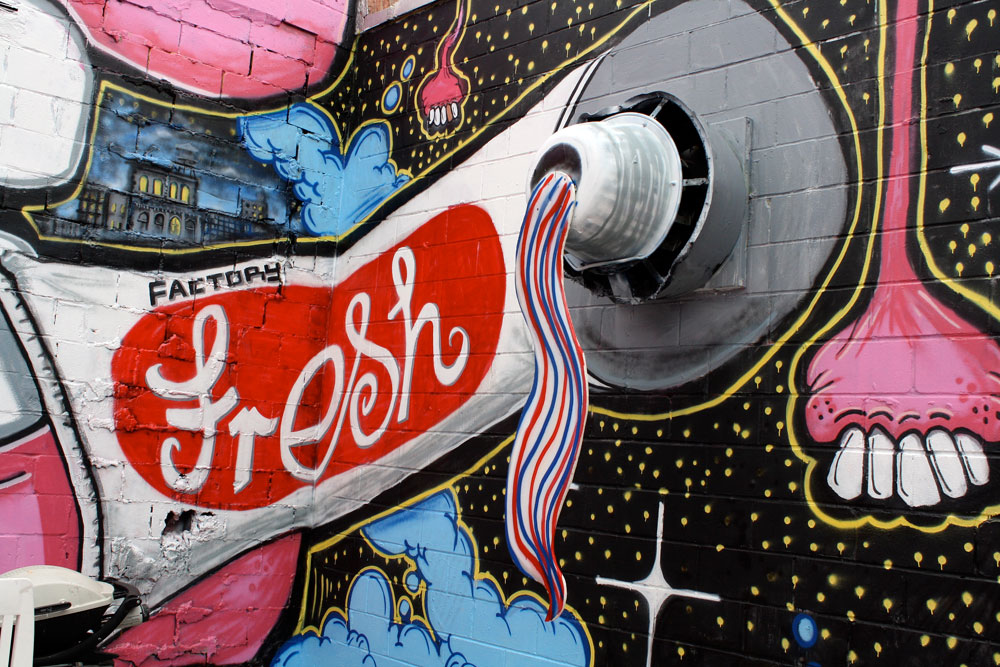This intriguing graffiti art is a captivating 3D mural painted on the exterior of a building, creatively integrating its ventilation system. The mural features a surreal night cityscape reminiscent of a Van Gogh painting, with a black sky dotted with stars and swirling blue clouds. The central element is a giant toothpaste tube adorned with the label "Factory Fresh" set against a vivid, oval-shaped red background. The multicolored toothpaste – in shades of white, blue, and orange – appears to flow out of the building's ventilation system, giving the artwork a sculptural, lifelike quality. The scene is framed by abstract, elongated shapes resembling gums and teeth, alongside eerie buildings, all painted against black and pink walls, adding to the surreal and dynamic nature of the piece.